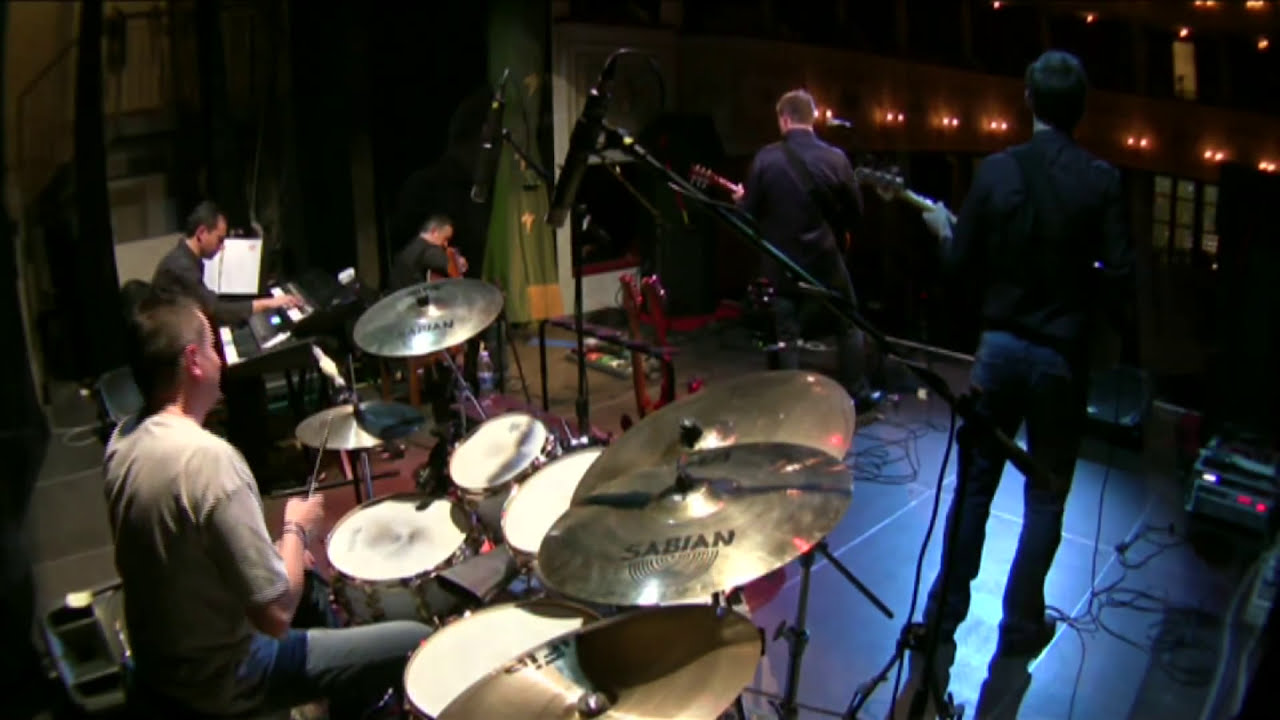This is a horizontal rectangular image capturing a band on stage from behind the lead performer, likely the singer. The image offers a view towards the darkened audience, barely visible due to insufficient lighting. Center stage is the lead performer, a slender man wearing jeans and a long sleeve shirt, playing a bass guitar. Directly to his left is a drummer, identifiable by a large drum set equipped with at least four drums and several cymbals. The drummer, with short hair and a beige t-shirt, holds his drumsticks mid-action. Behind the drummer, a pianist with dark hair is hunched over a dual-keyboard instrument. To the left of the stage, at the front, another man with gray hair, wearing a black shirt, is playing an acoustic guitar. The scene is bustling with stage equipment, wires, and dim lights focused towards the audience area, indicating the setting is a live concert.